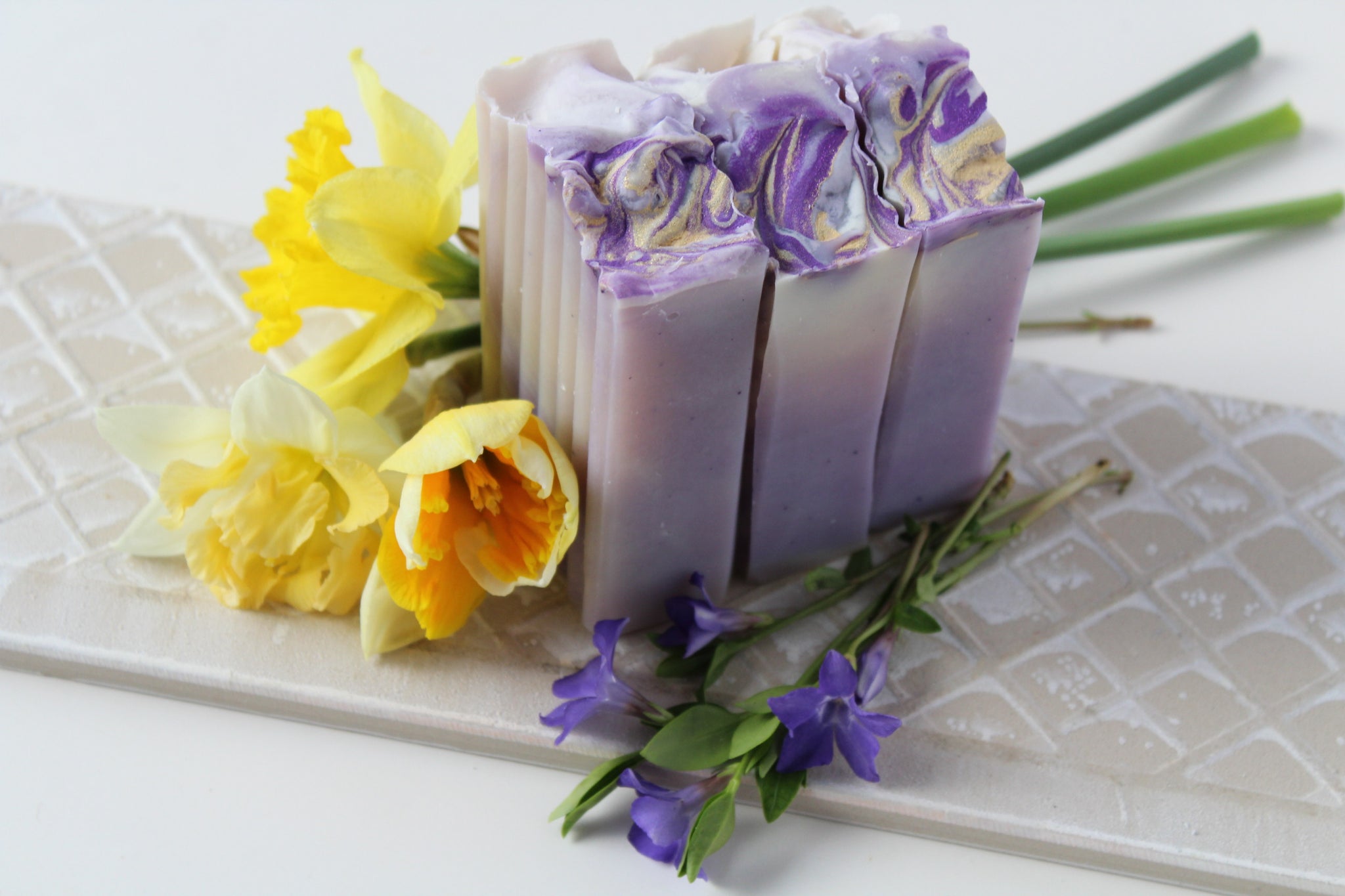This photograph, likely intended for an advertisement or a website, showcases three blocks of homemade soap arranged on a light tan tile with a subtle diamond pattern. The soap blocks are standing upright, each featuring a textured front with ridges and a beautifully marbled top. The tops display an intricate swirl of colors, including dark purple, lavender, white, and touches of gold, resembling melted ice cream in their fluidity. The sides and front of the soap blocks are predominantly purplish-gray with some variation in shading.

Accompanying the soaps are vibrant flowers that enhance the composition. In front, there are several purple flowers with green stems, adding a delicate touch of nature. Behind the soap blocks are three striking yellow flowers, which are likely hibiscus, providing a cheerful contrast to the cooler tones of the soap. All these elements are meticulously arranged on the textured tile, creating an appealing and harmonious display.